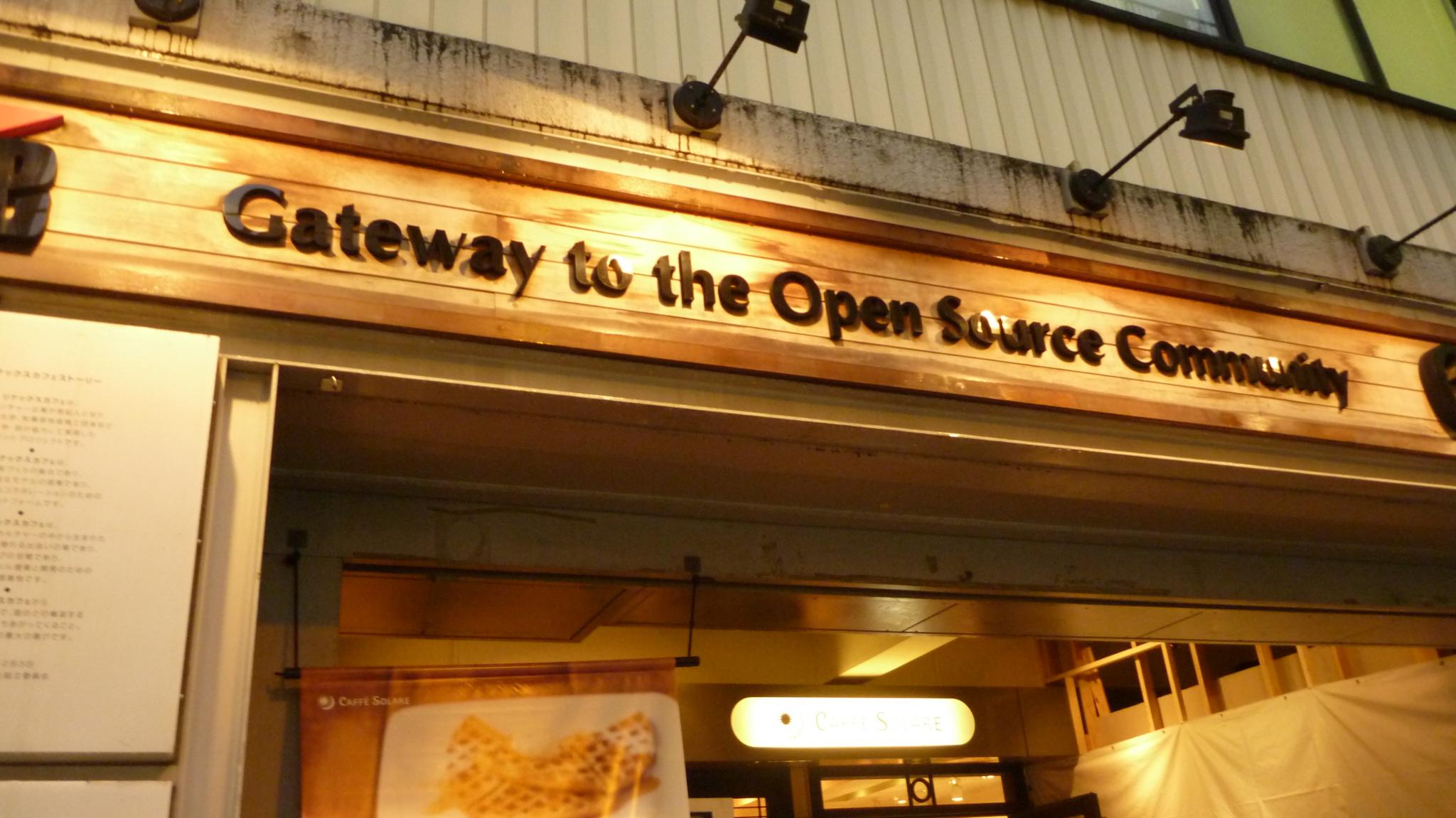This landscape-oriented color photograph depicts the front of a tan building, focusing primarily on a horizontal, wooden canopy sign with a rich oak finish. The sign prominently displays the text "Gateway to the Open Source Community" in bold, black lettering. Above this sign, there is a row of protruding lights attached to a section of corrugated metal in white and gray, designed to illuminate the storefront. 

On the facade, to the left of the entrance, a reader board with a white background features several lines of black writing, though the text is too blurry to decipher. Below the sign, partially visible, is a double door with black frames, hinting at an open doorway. The interior is warmly lit, casting an orange glow. Close-up, an additional sign or possibly a menu poster is visible, adorned with an image of waffles topped with syrup and butter, further suggesting the varied offerings within. A light fixture hangs just above the door, casting additional illumination on the entryway.